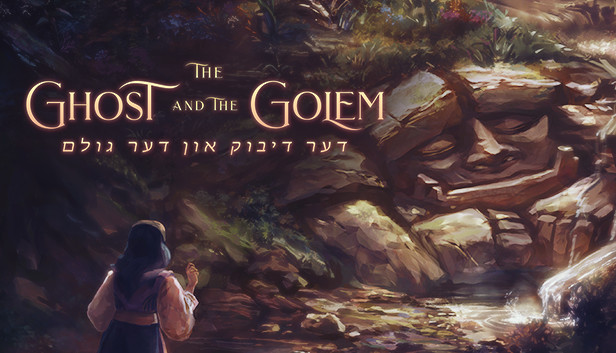The image depicts a detailed artwork that appears to be a promotional poster for a movie, titled "The Ghost and the Golem," written in gold letters in the top left corner, followed by foreign, possibly Hebrew, script. Dominating the scene is a rocky hillfront sculpted to resemble the imposing face of a giant, with two large rocks forming the eyebrows, a prominent nose, closed eyes, and a broad mouth, as well as arms extending down to the ground, seemingly embracing a pond. The rocky figure is set against a backdrop adorned with greenery and vibrant blue and pink flowers. In the foreground, a woman with dark hair and her back turned to the viewer stands in a white blouse and possibly dark purple bottoms. She is gazing towards the stone figure, her arm raised slightly as if reaching out. The scene captures an intriguing blend of natural and fantastical elements, enriching the enigmatic ambiance of the artwork.